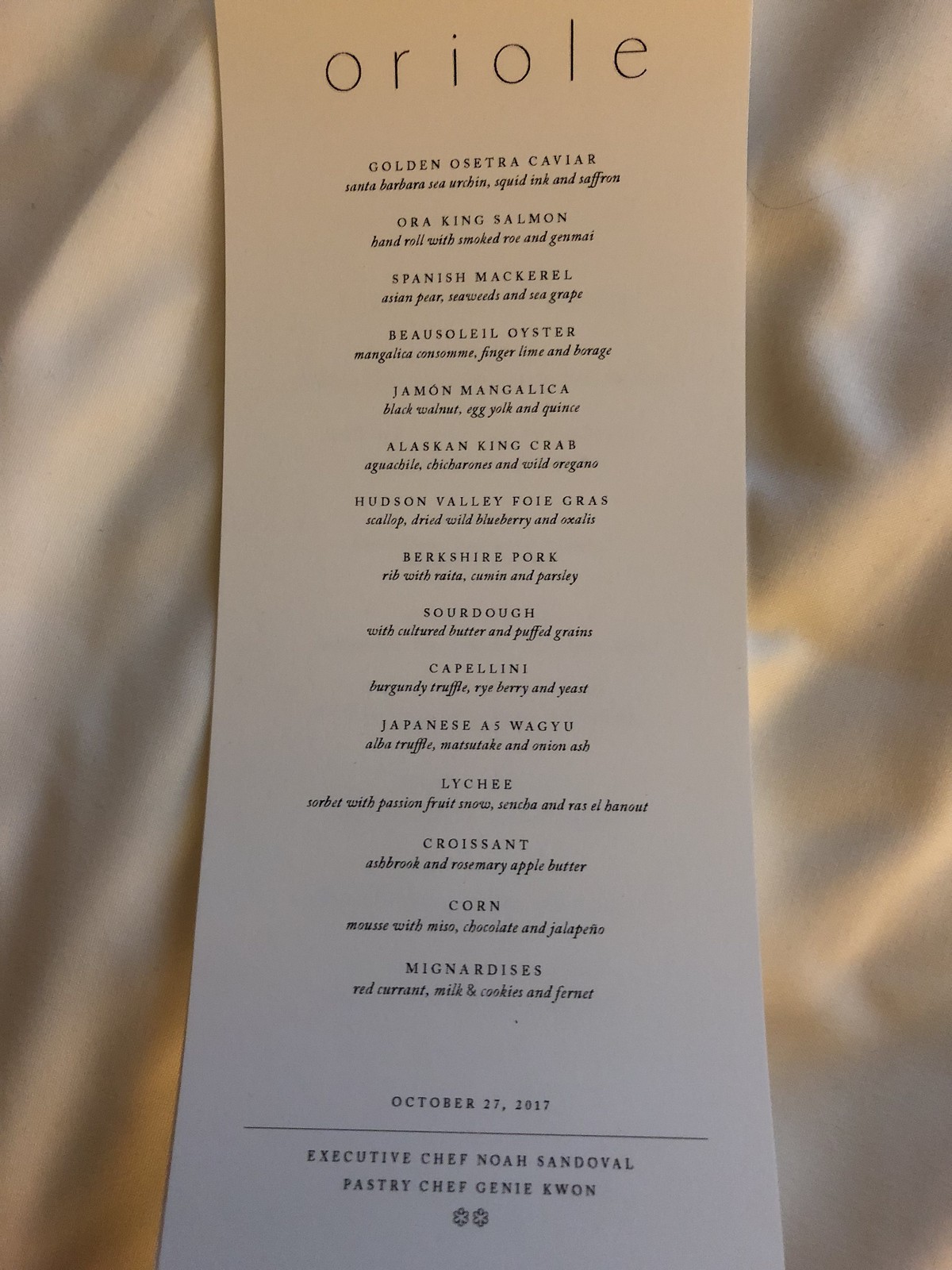Close-up image of a meticulously designed menu printed on high-quality white cardboard, featuring a long rectangular shape. At the top, the menu prominently displays the name "Orioli" in large, elegant print. The menu lists various gourmet items, including Golden Osetra Caviar, Aura King Salmon, Spanish Mackerel, Busulil Oyster, Jamon Mangalica, Alaskan King Crab, Hudson Valley Foie Gras, Berkshire Pork, Sourdough, Capellini, Japanese Wagyu, Lychee, Croissant, Corn, and Magnadise. The date for this exquisite dining experience is noted as October 27th, 2017. At the bottom of the menu, the names of the culinary maestros are inscribed: Executive Chef Noah Sandoval and Pastry Chef Jeannie Kwan.